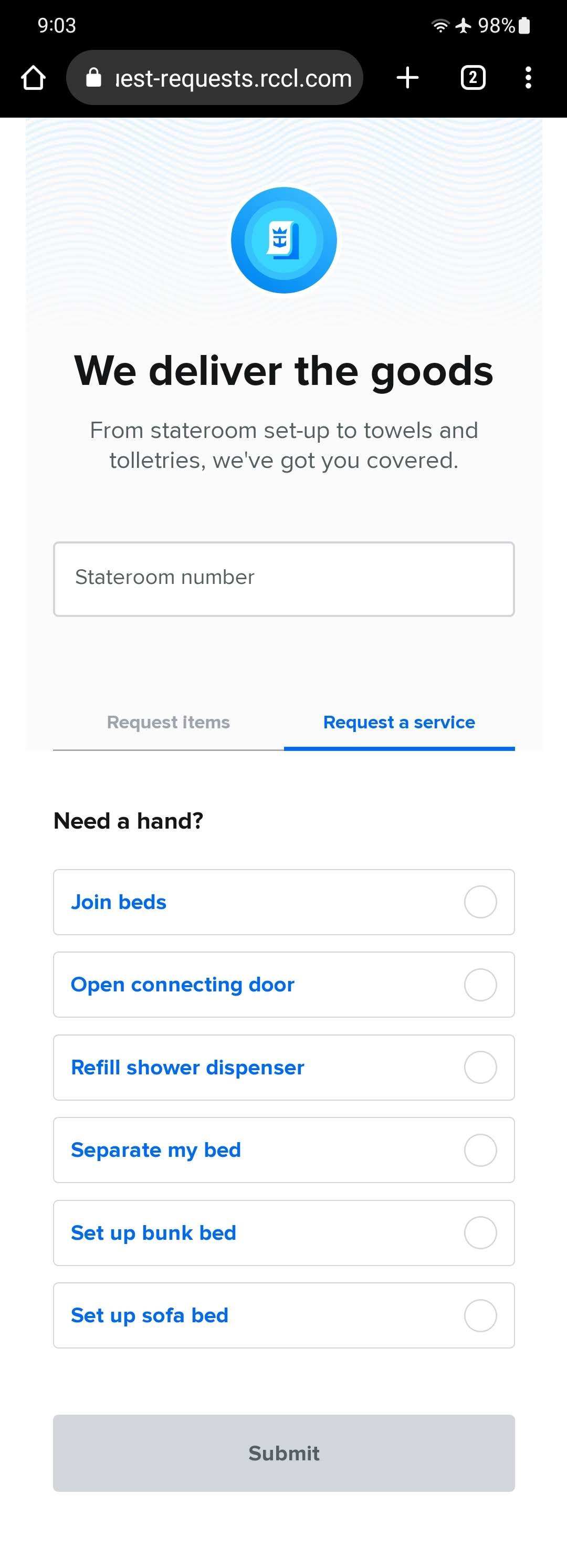This is a detailed screenshot of a delivery service interface, likely associated with a hotel or cruise line. At the top of the page, a black banner features several elements: a home icon, a search bar displaying "request.rccl.com," a plus symbol for adding an additional tab, a notification that we are currently in tab 2, airplane mode indicator, a 90% battery icon, and a menu represented by three dots.

Directly beneath the black banner is a blue circle with a blue background, featuring a white paper icon. On this paper, there is a blue crown above a blue anchor, symbolizing the brand's identity. Below this emblem, in bold black letters, it reads "We Deliver the Goods." Further description in smaller text highlights the range of services offered: "From stateroom setup to towels and toiletries. We've got you covered."

A rectangle box labeled "Stateroom Number" is situated below this description, presumably for user input. Two adjacent tabs allow users to choose between "Request Items" and "Request a Service."

Beneath these tabs, a heading in black letters, "Need a Hand?" precedes six selectable options, each printed in a white background with blue text, accompanied by a circular checkbox on the right:

1. Join beds
2. Open connecting door
3. Refill shower dispenser
4. Separate my bed
5. Set up bunk bed
6. Set up sofa bed

At the bottom of the interface, a "Submit" button allows users to finalize their requests. This image appears to depict a user-friendly app designed to cater to guest needs, enhancing their in-room experience.